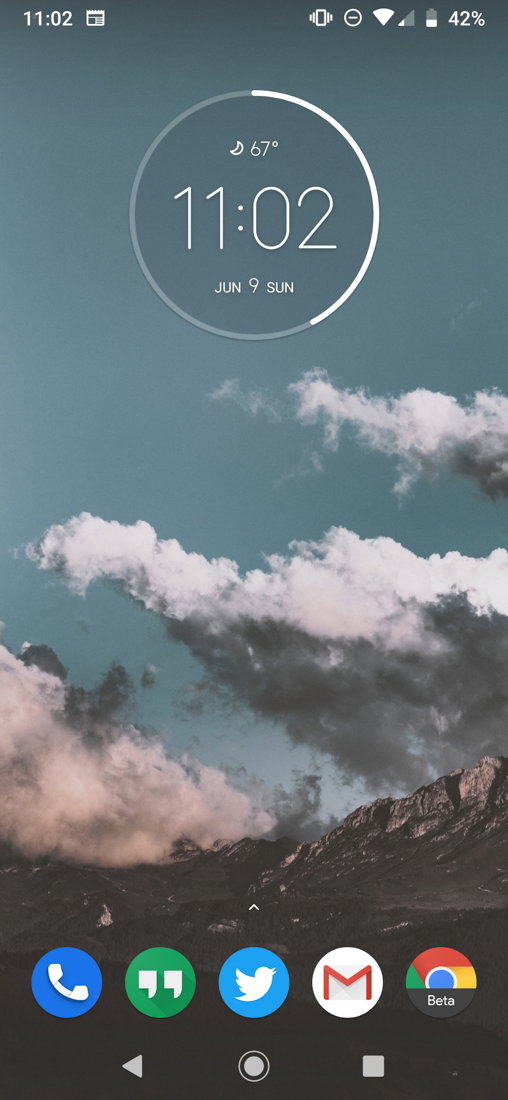In this detailed screenshot of a mobile device’s home screen, the time is prominently displayed at the top left corner, showing 11:02. The status bar is populated with various icons, including a newspaper icon, phone vibration icon, do not disturb icon, a full WiFi signal strength icon, network signal icon, and a battery indicator displaying just 2% remaining. The weather information indicates a temperature of 67 degrees Fahrenheit. Just beneath this, the date is clearly shown as Sunday, June 9.

The bottom of the screenshot showcases a row of frequently used applications: the Phone app, Google Hangouts, Twitter, Gmail, and Google Chrome. Below these apps, the navigation keys for back, recents, and home are visible. This detailed depiction reveals a well-organized home screen with essential information and quick access to key applications.